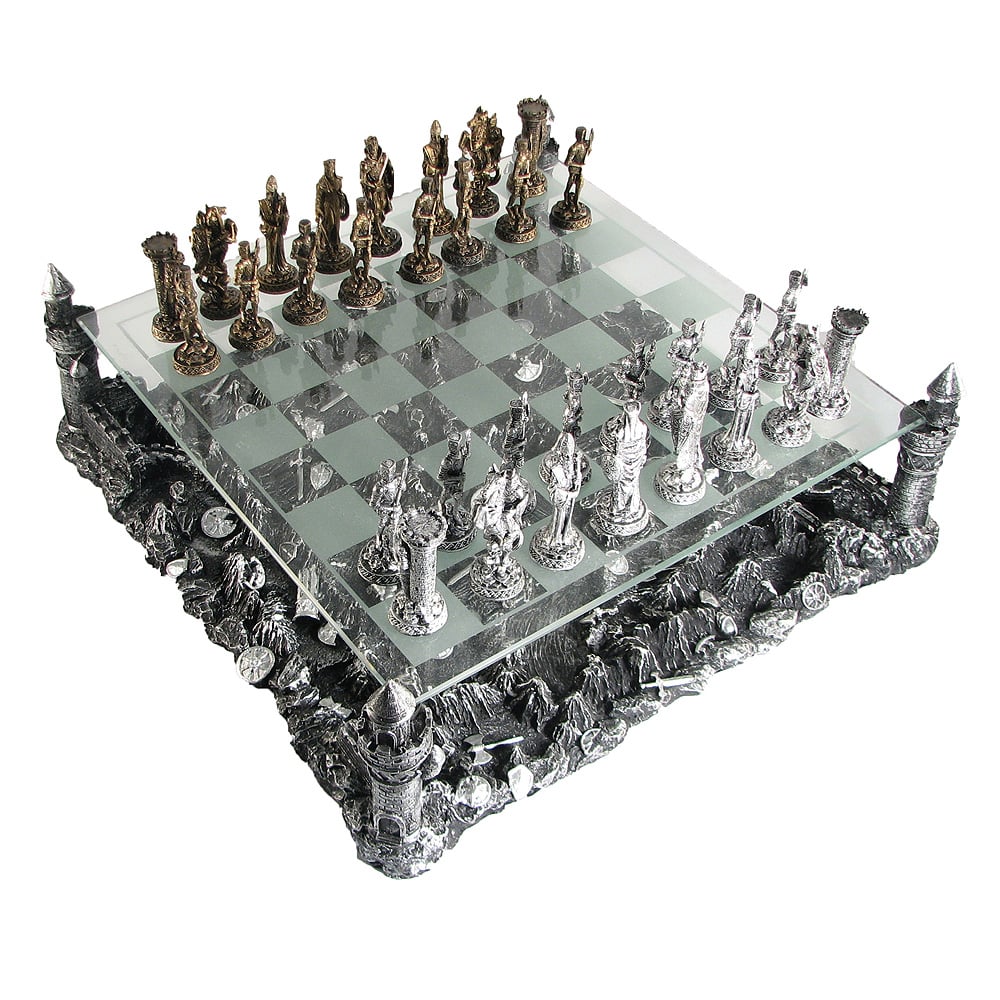The image showcases a highly ornate and luxurious chess set, meticulously arranged on a pristine white surface with a white background to emphasize the product. The chessboard itself is a clear green checkered glass square composed of 64 smaller squares. This elegant board is supported by an intricate pewter base designed to resemble a mountainous battleground, complete with intricately carved weapons. Each of the four corners of this pewter base is adorned with towering castle structures that elevate and support the glass board above. The chess pieces, positioned in classic formation, are distinguished by their colors and elaborate designs resembling knights, warriors, kings, and queens. The pieces on the upper left side of the board, facing toward the viewer, are gold-colored, while those on the lower right side, facing away from the viewer, are silver-colored. The entire setup gives an impression of floating due to the clean, isolated background, highlighting the chess set's artistic and potential material value, including speculation of genuine gold and silver elements. The photograph, captured in a square format, aligns the board diagonally to the viewer, enhancing the visual appeal and emphasizing the exquisite craftsmanship and opulence of the chess set.